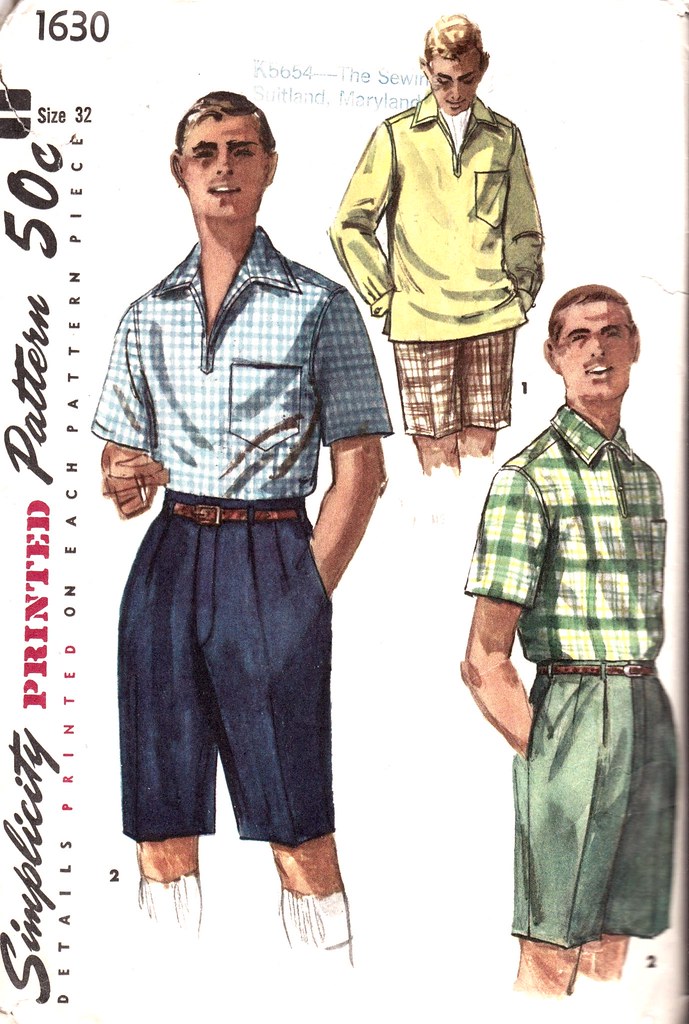The cover of this vintage Simplicity Printed Pattern, priced at 50 cents, features a detailed illustration of three men modeling different outfits. On the left-hand side of the envelope, the words "Simplicity Printed Pattern" are vertically arranged in a mix of script and stencil font, with "50 cents" listed. Above the label, the pattern number "1630" is prominently shown, with "size 32" indicated horizontally below it. Underneath the Simplicity label, it states "Details Printed on Each Pattern Piece" vertically.

In the top center, there's a slightly faded stamp mentioning "Maryland." The illustration depicts three white males, each facing forward and dressed in varied outfits suitable for warm weather. The first man wears a yellow popover shirt over brown plaid pants, the second man sports a blue checkered short-sleeve shirt with long navy Bermuda shorts, and the third is dressed in a green and yellow plaid shirt over pleated green Bermuda shorts. Two of the men have their hands in their pockets. The illustration appears to be rendered in either colored pencil or watercolor, enhancing the vibrant details and textures of the clothing patterns.